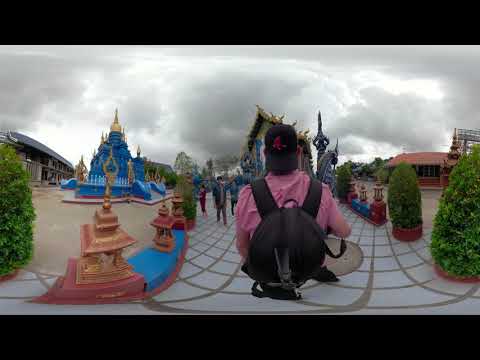This panoramic photo captures a young man crouching on a white stone tile path, surrounded by an ornate temple landscape. Seen from behind, he sports a backwards black baseball cap emblazoned with a large red 'A' and a short-sleeved pink (or purple) shirt. A black backpack with two straps is secured over his shoulders, possibly rigged with a selfie stick. The scene around him features multiple conical bushes and brown lanterns flanking the path. To the left stands a highly decorative, blue and gold statue resembling a miniature palace. This statue is part of a vibrant and colorful temple complex, which includes other buildings with gold elements, although some details are obscured by the man's position. The setting, likely in an Asian country, displays the typical architecture of a Buddhist temple with spires and additional structures, creating a richly detailed and culturally immersive backdrop. The overcast sky adds a subdued cast to the otherwise lively scene.